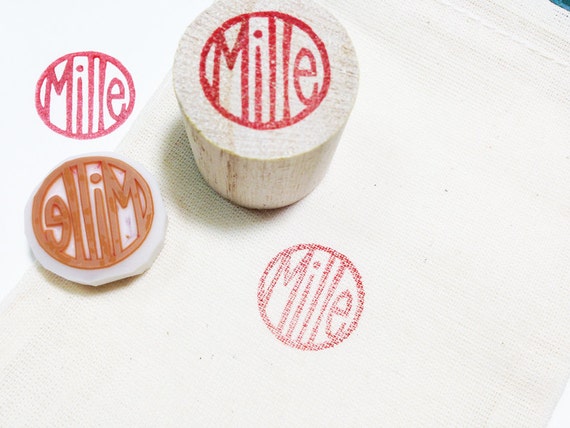This detailed image features a circular wooden stamp prominently embossed with the word "Mille" in tall, red letters that fit neatly within a red circular border. The composition includes multiple views: the stamp itself positioned towards the left side of the closely-cropped frame, a photo showing the stamped image in red ink on a white background, and another example printed on a textured, ribbed white surface, possibly fabric or thick paper. The stamp, shaped like a straight-sided barrel and reminiscent of a wide cork, is crafted from a white wood with a rubberized bottom where the reversed letters of "Mille" are visible. The consistent colors throughout the image are red and white, with the natural wood hue adding a subtle contrast. There is no other text present, and the background, a clean white or beige canvas, highlights the stamp’s details clearly.